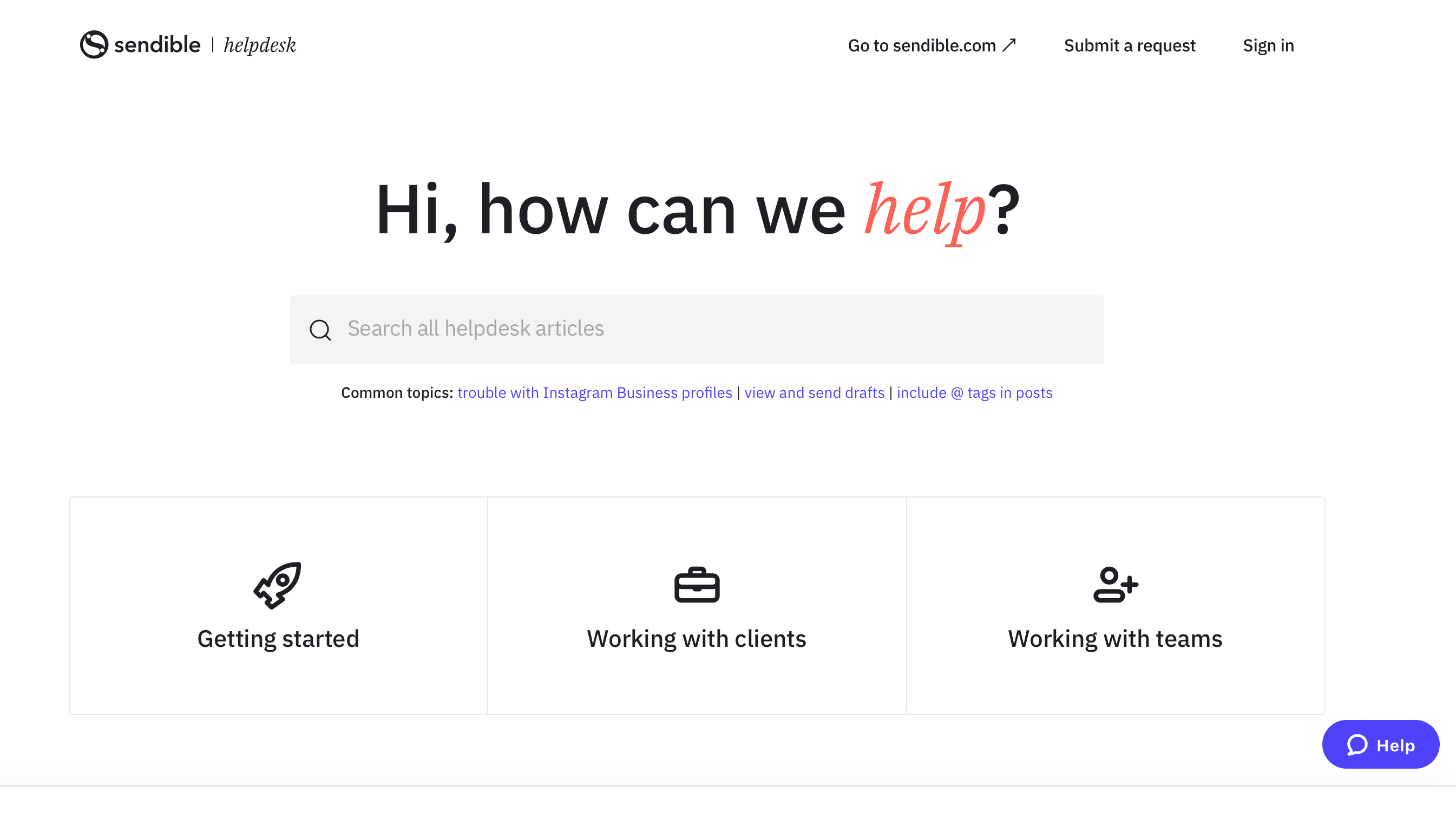The screenshot showcases the help desk webpage of a website called Sendible (spelled S-E-N-D-I-B-L-E). The Sendible logo, a circle featuring a squiggly line, appears prominently. The page title reads "Sendible | Help Desk," formatted with a vertical pipe symbol. On the right side of the page, navigation options include "Go to sendible.com," "Submit a request," and "Sign in."

Central to the page is a large welcoming text stating "Hi, how can we help?" with the word "help" highlighted in red italics, contrasted against a black sans-serif font for the rest of the text. Directly below this text is a search box accompanied by a magnifying glass icon and placeholder text reading "search all help desk articles."

Further down, a list of common topics is presented, including "Trouble with Instagram business profiles," "View and send drafts," and "Include @ tags in posts." At the bottom of the page are three large, white, rectangular buttons, distinguished by a light gray border. These buttons feature specific icons and text: the first button, marked with a racket icon, reads "Getting Started"; the second, with a briefcase icon, says "Working with Clients"; and the third, displaying an icon of a person's upper torso with a plus sign, states "Working with Teams."